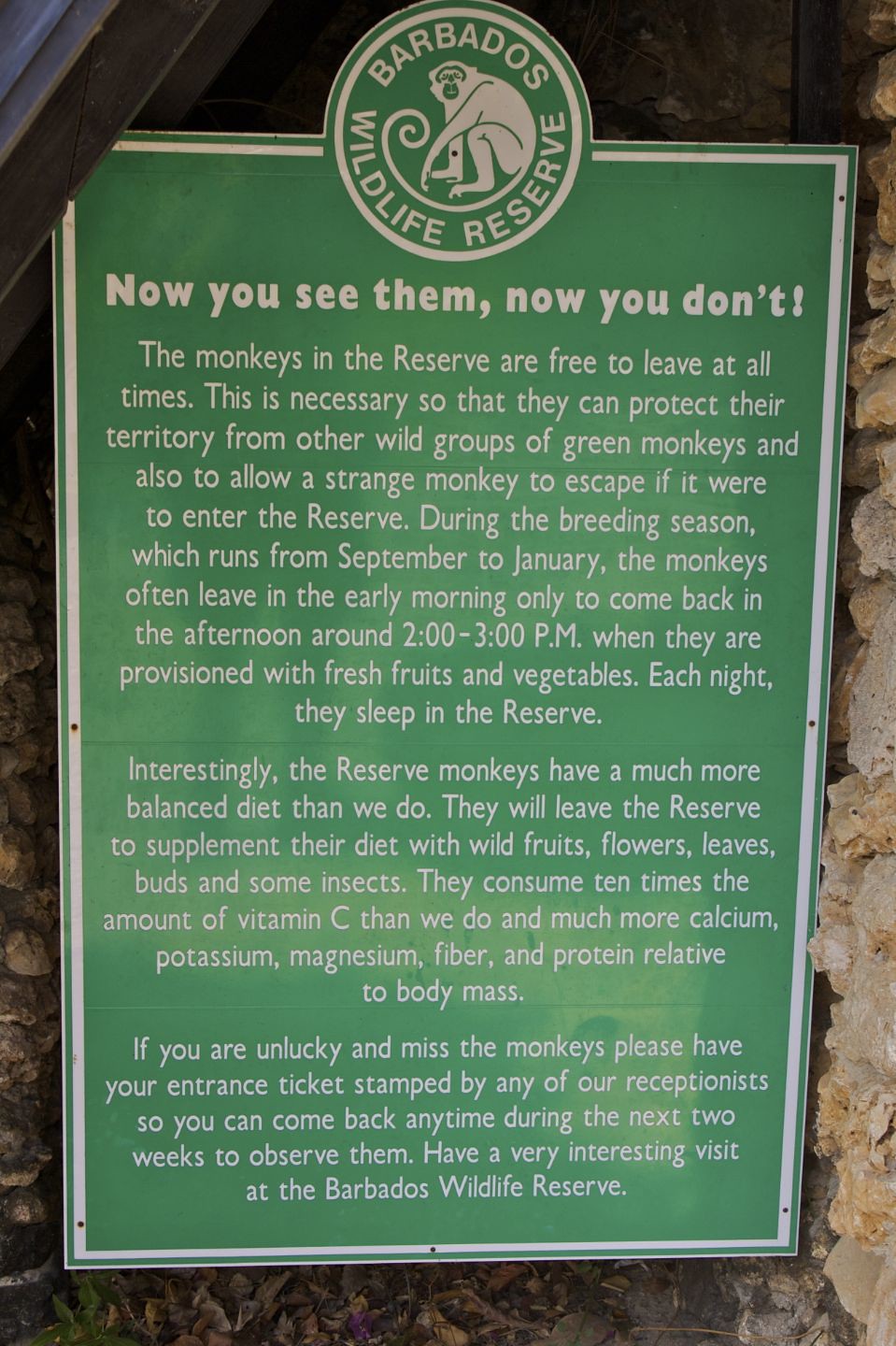This is a detailed color photograph of an informational sign taken outdoors during the daytime. The sign is mounted against rocks and surrounded by leaves. It has a green background with a white border and a white circular emblem at the top. Inside the circle is a picture of a monkey, along with the words "Barbados Wildlife Reserve" in white typography. Beneath this emblem, the sign prominently displays the headline "Now You See Them, Now You Don't." The text below the headline is organized into three paragraphs, which describe the behavior and habits of the monkeys in the Barbados Wildlife Reserve. 

The sign explains that the monkeys are free to leave the reserve at all times to guard their territory against other wild groups and to allow any strange monkeys to escape if needed. It is noted that during the breeding season, from September to January, the monkeys often leave in the early morning and return around 2 to 3 p.m. when they are provided with fresh fruits and vegetables. At night, they sleep in the reserve. The monkeys have a diet more balanced than humans, supplementing their meals with wild fruits, flowers, leaves, buds, and some insects, consuming significantly more vitamin C, calcium, potassium, magnesium, fiber, and protein relative to their body mass. Additionally, if visitors miss seeing the monkeys, they can have their entrance ticket stamped by a receptionist, allowing them to return within the next two weeks to observe the monkeys. The overall style of the photograph is representational realism, capturing the detailed text and imagery on the sign with clarity.